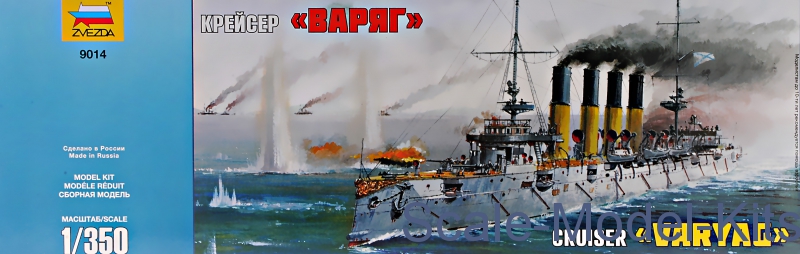The horizontal, rectangular image appears to be a detailed poster or the top of a model kit box, featuring an artistic rendering of a battleship. The ship, presumably named "Cruiser Varvala," is depicted sailing on blue water. The battleship is a long and narrow vessel equipped with four central smokestacks billowing black smoke and a prominent tower at the front, likely the bridge from where the ship is steered. Surrounding the primary ship, there are multiple explosions in the water, suggesting an active battle scene. Behind the cruiser, several more ships are visible in the distance, also emitting smoke, some appearing to be on fire or hit by bombs. Above and beside the image, text in white lettering includes "Model Kits, Cruiser Varyal," and a logo that reads "Zvezda," indicating a scale model, possibly "1:350" and "Made in Russia." The poster is visually striking, combining elements of detailed ship construction with dynamic action, suggesting it is part of a model kit packaging designed to attract enthusiasts with its vivid and dramatic depiction of naval warfare.